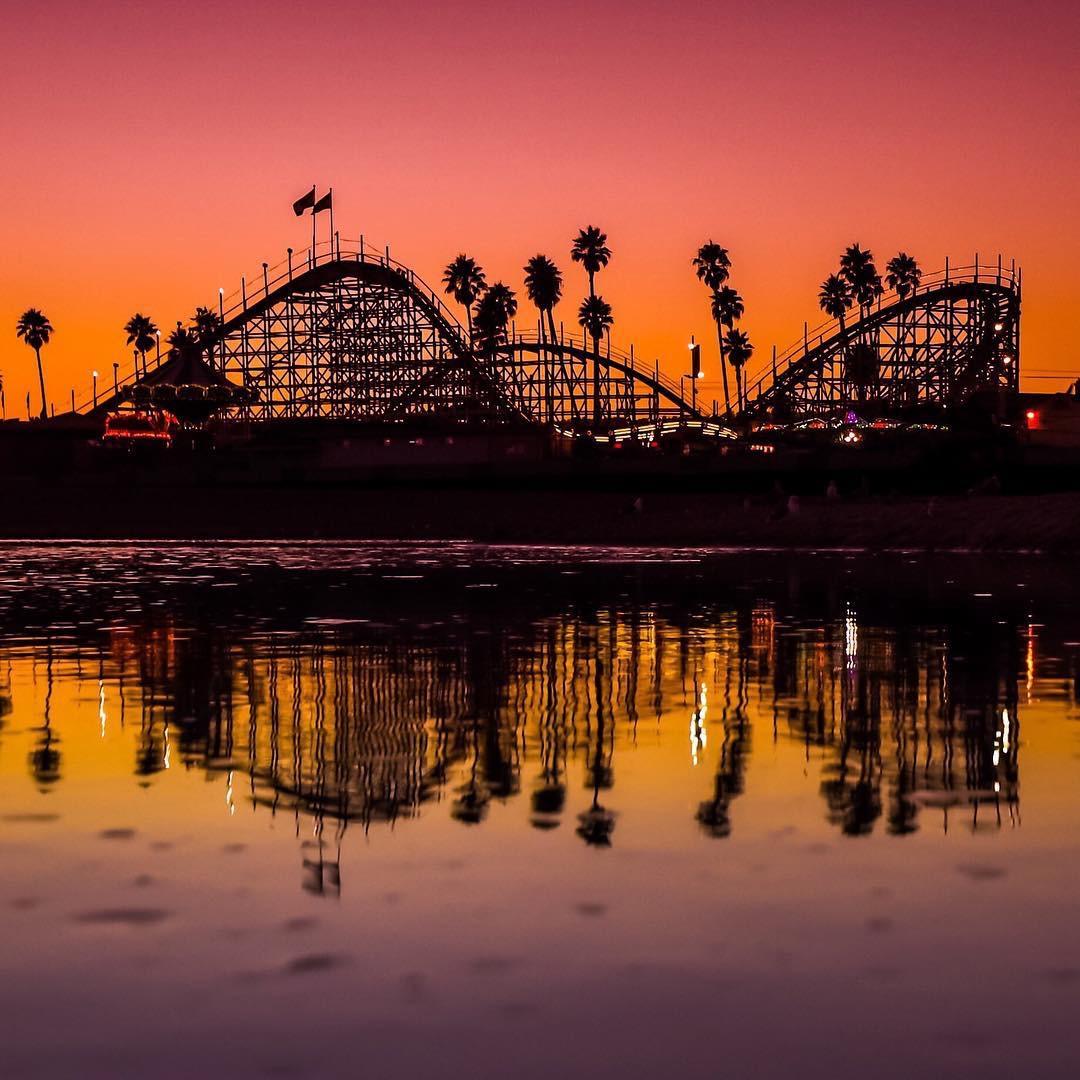In this captivating evening scene, a silhouetted roller coaster stretches across the horizon, likely part of a theme park near water, possibly in Santa Monica. The roller coaster, with its undulating dips and curves, features a prominent tall peak on the left adorned with flags, a shorter hill in the middle, and a sweeping curve on the right. Palm trees frame the roller coaster, their dark forms complementing the silhouette against the sky. The gradient sky transitions from a pinkish hue at the top to a deep orange near the horizon, reflecting beautifully in the calm water below. The water mirrors the dark silhouette of the roller coaster and the vibrant sky, with a shimmering effect from the scattered lights along the ride. The reflection in the water shifts from dark black in the distance to a murky gray to a warmer orange closer to the viewer, capturing the serene yet dramatic essence of sunset.